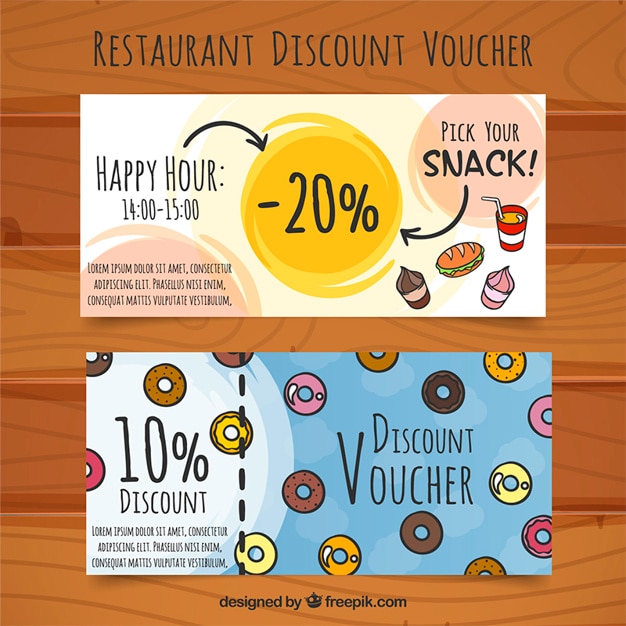The image features a visually attractive ad with two restaurant discount vouchers displayed against a digitally created wood-paneled background, colored to resemble reddish-brown wood. At the top, there is bold black text that reads "Restaurant Discount Voucher." 

Below the title, the first voucher appears as a rectangular ticket promoting a "Happy Hour" offer from 14:00 to 15:00. It prominently offers a 20% discount on snacks, accompanied by intricate arrow graphics connecting different circles highlighting the discount and selection option. The voucher is adorned with illustrations of various snacks, including a sandwich with green lettuce, a red-and-white cup with a bendy white straw filled with an orange drink, and possibly a chocolate cupcake and a vanilla cupcake with a pinkish frosting.

Underneath the Happy Hour offer, there's a second blue voucher labeled "10% Discount Voucher." This contains an array of colorful donuts with different frostings and designs, including brown, pink, yellow, and speckled varieties, some featuring sprinkles. The background here showcases donuts in a visually appealing scattered pattern. Both vouchers have "Lorem Ipsum" placeholder text at the bottom and feature a watermark that says "designed by freepik.com," with a logo of a black crown situated between "by" and "freepik."